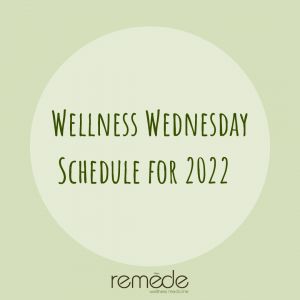The image features a design primarily in shades of green, with a square-shaped outer border in a darker green hue. Inside this square, there is a prominent light green circle. Centered within this circle, in dark green uppercase letters, is the text "WELLNESS WEDNESDAY." Beneath this headline, about two inches down, is another line of dark green text reading "Schedule for 2022."

Below the light green circle, there is the word "REMEDE," with a small diacritical mark above the second 'E,' possibly indicating the pronunciation "Remedy." The overall design employs varying shades of green, with the text in a deep evergreen shade, providing a harmonious and cohesive look.